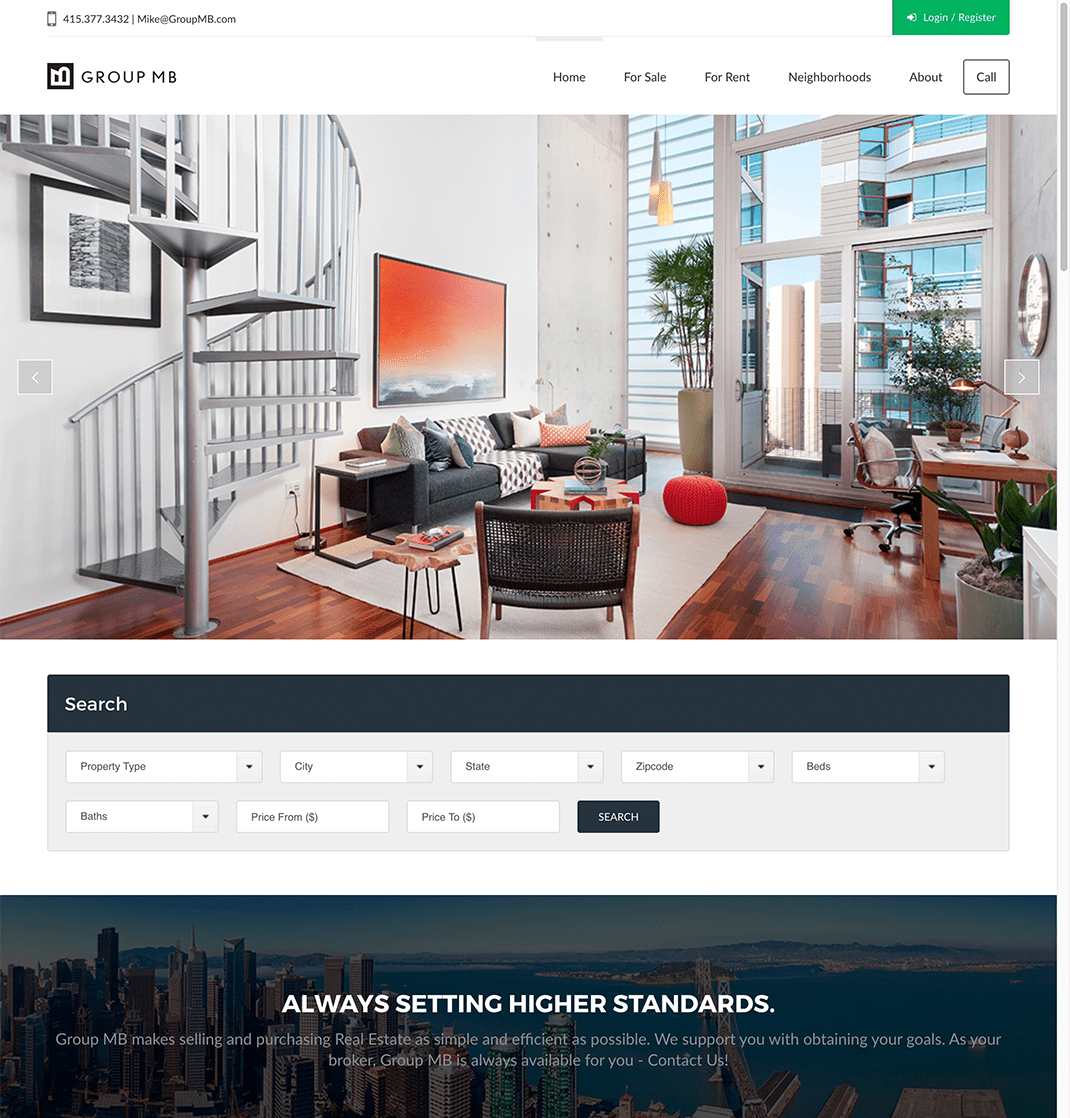The image showcases the homepage of a real estate website called Group MB, which features a variety of properties available for sale. At the center of the screen is a prominent image of a stylish designer apartment. This apartment boasts an elegant aluminium glass spiral staircase as its focal point. The interior is tastefully decorated with paintings adorning the walls, a cozy settee, and a very large window that offers a view of an adjacent apartment building. The room features pristine wooden flooring accentuated by a soft rug, and it is furnished with a small central table as well as another table equipped with an office chair and a lamp overhead.

Below this central image is a grey panel labeled "Search," where users can refine their property search by specifying details like property type, city, state, zip code, number of bedrooms, number of bathrooms, and price range (with both an upper and lower limit). To complete the search, users can click the "Search" button.

At the very bottom of the screen, there is another panel displaying an image of tower blocks forming a cityscape overlooking a body of water, possibly a lake. Directly above this cityscape image is the website’s tagline: "Always Setting Higher Standards."